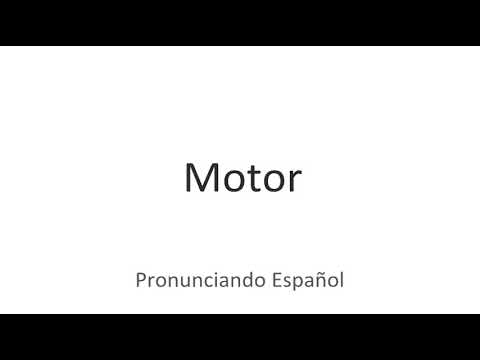This image appears to be a screenshot featuring text on a primarily white background. It has thin, solid black borders at both the top and bottom, giving it a widescreen appearance. Centered in black, bold text is the word "Motor" with a capital 'M'. Directly below this, in a smaller, grayer font, is the Spanish phrase "Pronunciando Español," suggesting that this might be related to a translation or language learning tool. The simplicity of the layout highlights the emphasis on the textual content against the minimalistic design.